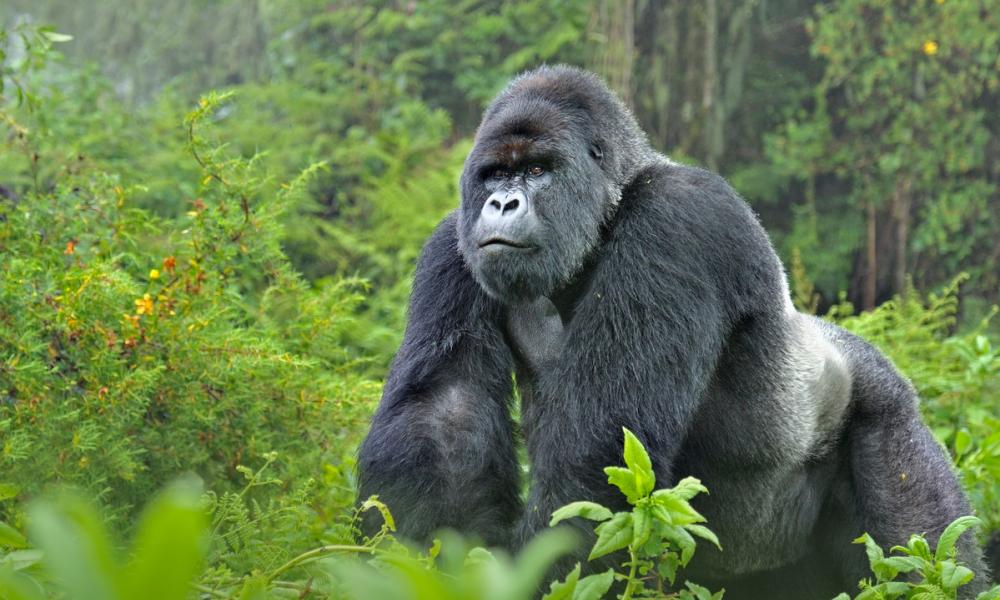A professional full-color photograph captures a majestic silverback gorilla in its natural jungle habitat, using natural daylight. The image, rectangular and horizontally aligned, presents a close-up of the large male gorilla, showcasing his dark brown and black fur interspersed with silver patches on his back and sides. The gorilla, standing on all fours, is framed by dense, vibrant greenery with an abundance of tall weeds, stems with small leaves, and a few yellow and red flowers, particularly noticeable towards the center left of the image. His face displays a mix of white around the nose and a hint of brown above his eyes. The backdrop is a lush forest with a blurry array of thin tree trunks and thick foliage, entirely free from any clear ground. Sunlight filters through, illuminating the gorilla's robust frame and adding a natural glow to his imposing presence. The overall scene breathes life, fully immersing the viewer in the untamed beauty of an unspoiled jungle.